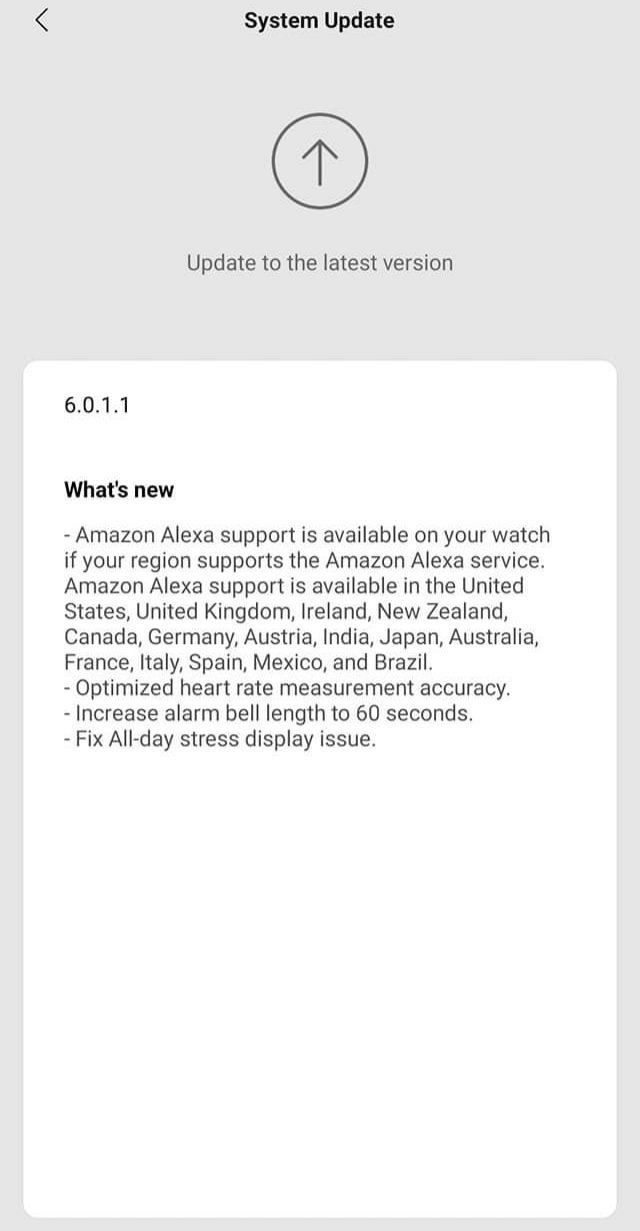Captured from a cell phone screen, this image prominently shows a system update notification. At the top, a message reads "System Update" accompanied by an arrow within a circle, indicating an update to the latest version. Further down, in a large white rectangular box, the new version number "6.0.1.1" is displayed. Below this, the update details begin with "What's New" and specify that Amazon Alexa support is now available on the user's watch, provided their region supports the service. The regions mentioned include the United States, United Kingdom, Ireland, New Zealand, Canada, Germany, Austria, India, Japan, Australia, France, Italy, Spain, Mexico, and Brazil. Additionally, updates include optimized heart rate measurement accuracy, an increased alarm bell duration to 60 seconds, and a fix for the all-day stress display issue. The interface features a gray background with blank spaces flanking the descriptive content, and a white foreground for the main information.